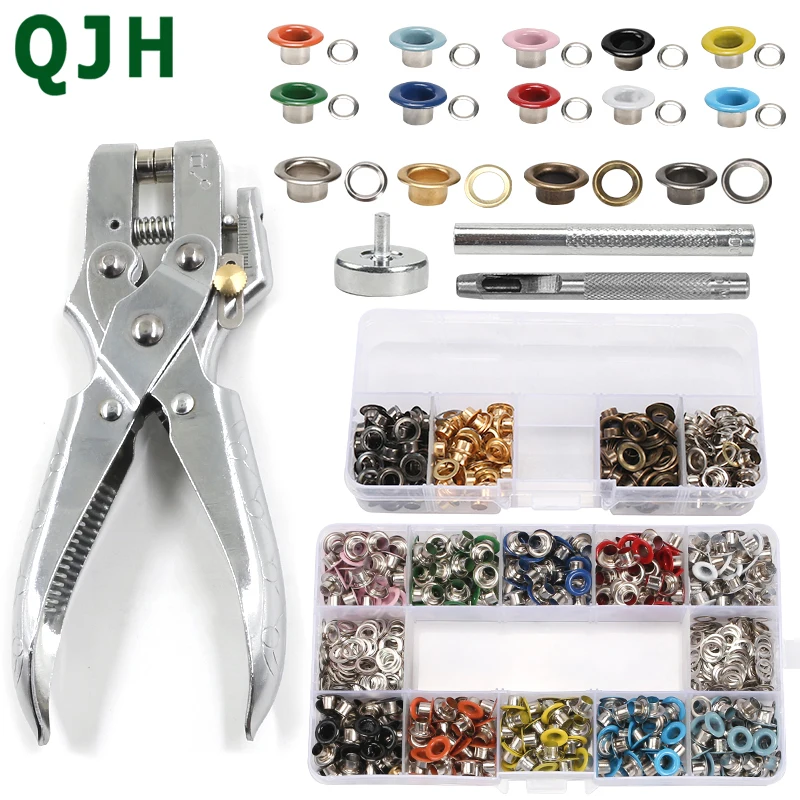The image depicts a rivet or button setter kit, which includes various components and tools. On the upper-left corner, the text "QJH" is written in green, likely indicating the brand. At the left side of the image, there is a silver, mechanical, hand-operated device resembling pliers or a hole puncher, equipped with a spring and cylindrical attachments, possibly used for setting rivets or buttons onto surfaces, such as fabric. The device also features a ruler-like measuring tool.

On the right side of the image, there is an array of colorful rivet pieces organized in rows, with colors including orange, green, blue, light blue, pink, red, black, white, yellow, chrome, gold, bronze, and silver. These rivet pieces are stored in a clear plastic container, which has compartments for each color, similar to a craft or fishing tackle box. The container ensures that all the small components are neatly sorted and easily accessible for use.